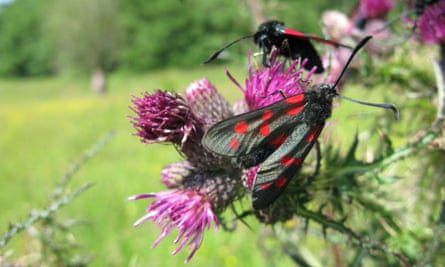In this vivid outdoor image, the focal point is a striking moth adorned with black wings and red spots, poised delicately atop a vibrant purple thistle flower. The intricate structure of the thistle is highlighted by its numerous strands and the thorny branch it's attached to, giving it a rugged appearance. Another moth, similarly marked, faces the central one, creating a sense of interaction. The soft-focus background features a blend of blurred trees and a hint of grass, enhancing the prominence of the foreground subjects. The lantern fly-like moths, despite their potential to cause significant ecological damage, add a striking contrast with their distinctive colors against the purple and green foliage.